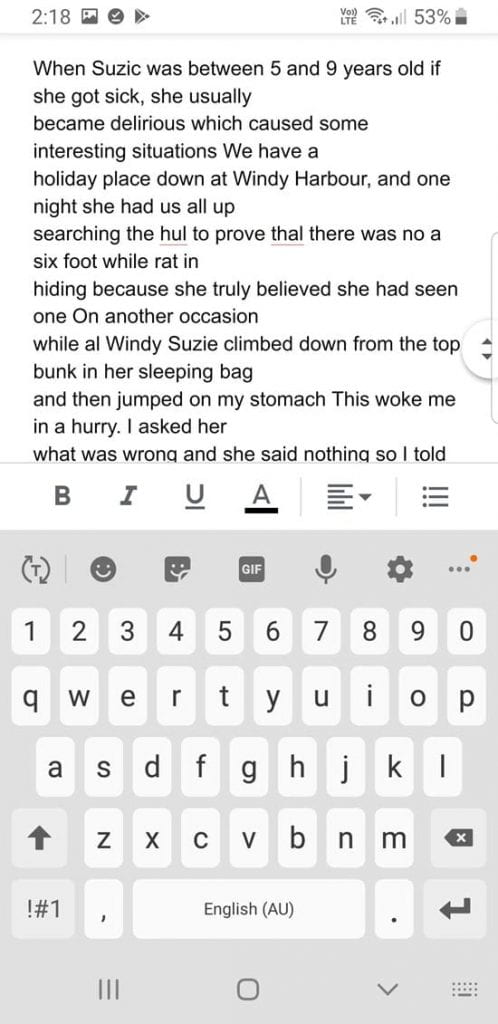A screenshot taken from an Android phone showcases a text message conversation. The background is completely white, blending seamlessly with the phone’s top toolbar. On the toolbar, the left side indicates the time as 2:18, while the right side shows the battery level at 53%, alongside several notifications on the status bar.

The focal point of the screenshot is the text message content displayed in the body. The bottom portion of the screenshot features the Android keyboard with a gray background and white keys. The message itself has some misspellings and reads, "When Suzik (spelled S-U-Z-I-C) was between five and nine years old, if she got sick, she usually became delirious, which caused some interesting situations. We have a holiday place down in Windy Harbor, and one night she had us all up searching the hole (spelled H-U-L) to prove thou (spelled T-H-A-L) there was not, there was no a six-foot white rat in hiding because she truly believed she had seen one on another occasion. While Al, Wendy, and Suzie climbed down from the top bunk in her sleeping bag and then jumped on my stomach. This woke me in a hurry. I asked her what was wrong, and she said nothing, so I told…" The message cuts off abruptly, leaving the narrative incomplete.